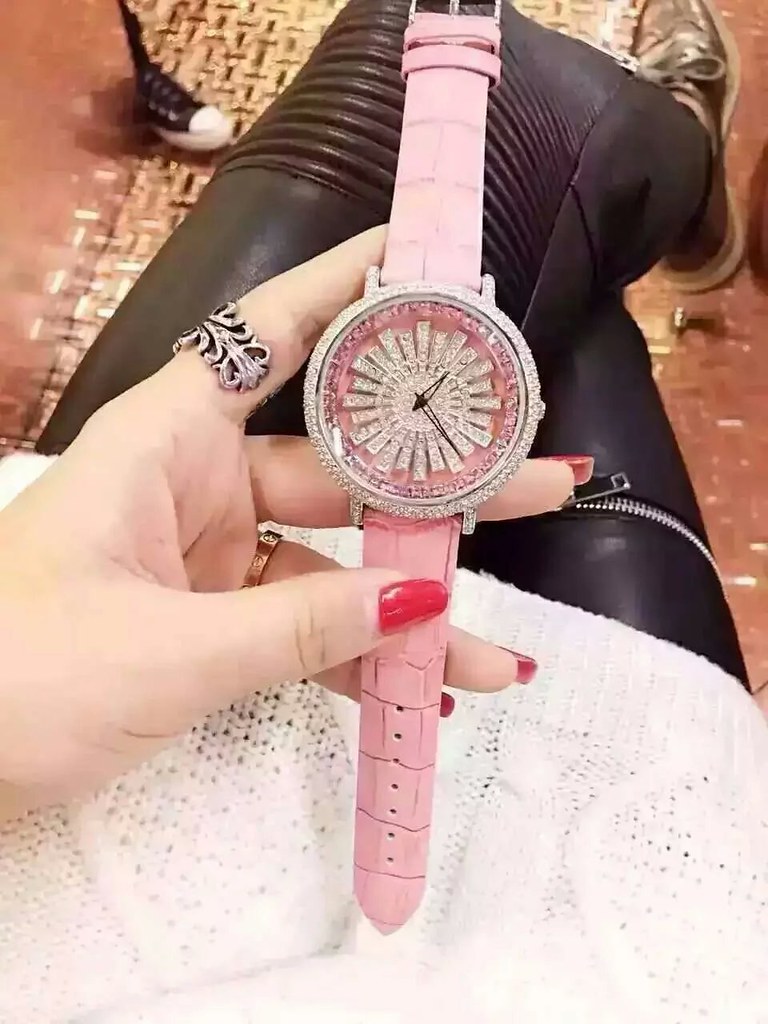In the image, a Caucasian woman is elegantly posed, showcasing a stylish ensemble and a luxurious accessory. She is dressed in a pristine white sweater paired with sleek black leather pants, which feature a distinctive silver zipper that runs horizontally across her right thigh. Her outfit is completed with a pair of striking gold shoes. Seated with her legs crossed, she has a confident and poised demeanor.

In her left hand, she holds an eye-catching pink watch. The watch boasts a vibrant pink band and a round face adorned with bezel-set diamonds or crystals, arranged in a starburst pattern. The watch face itself is pink, complemented by black hour and minute hands, and further embellished with pink stones around its border.

Accessorizing her look, the woman wears a silver filigree ring on her index finger and a gold ring on her ring finger. Her nails are beautifully painted in a pinkish-red shade, adding a touch of color to her overall presentation.

The setting of the photo includes a rustic brown floor with a gold mat on it. In the background, a black and white high-top tennis shoe, resembling a Converse sneaker, can be seen. This detailed image captures a moment of style and sophistication.